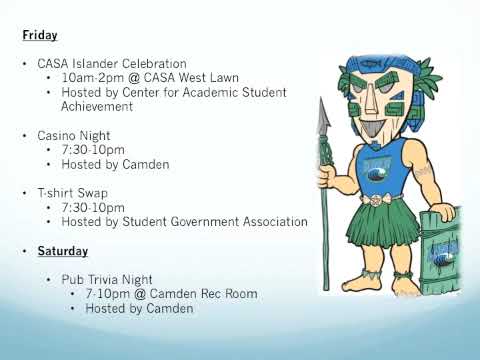In the image, a cartoon figure stands to the right, dressed in traditional attire reminiscent of ancient tribal cultures. The character wears a green grass skirt and a sleeveless blue tank top featuring an indistinct logo. A prominent wooden mask with white and green highlights, likely inspired by Amazonian or Mayan designs, adorns their face, along with a blue headband featuring a fish motif. The figure holds a green spear tipped with a pointed arrowhead in their right hand and a wooden shield in their left, both adorned with logos. The character also wears anklets on their bare feet.

To the left of the figure, text on a white and blue gradient background details an event schedule, resembling a PowerPoint slide or advertisement. On Friday, the events include the CASA Islander Celebration from 10 a.m. to 2 p.m. at CASA West Lawn, hosted by the Center for Academic Student Achievement; a Casino Night from 7:30 to 10 p.m., hosted by Camden; and a T-Shirt Swap from 7:30 to 10 p.m., hosted by the Student Government Association. Saturday's event is Pub Trivia Night from 7 to 10 p.m. at the Camden Rec Room, hosted by Camden.